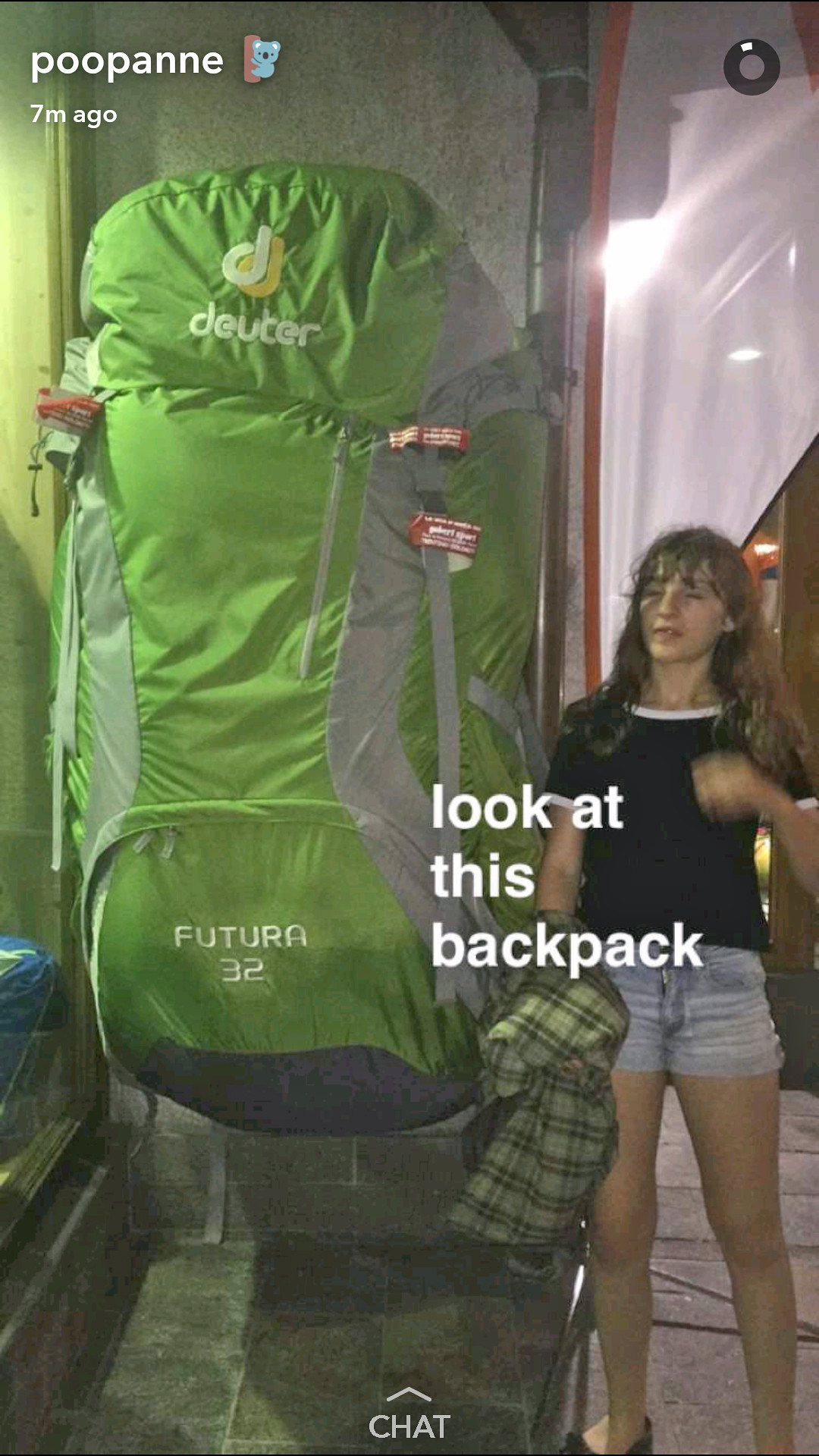In this rectangular vertical photograph, a young Caucasian girl with shoulder-length, dirty blonde hair is positioned on the right side of the image. She appears to be in her teens or early 20s, wearing a black shirt with blue jean shorts. Her left arm is in motion, and she is holding a green plaid shirt in her left hand. The girl stands next to an enormous green hiking backpack that dwarfs her; the backpack bears the "Deuter" logo with two overlapping 'D's, one white and one yellow. The backpack also has "Futura 32" written in white letters on the lower pocket, which is dark grey at the bottom, and grey stripes on its sides.

In the upper left-hand corner of the photo, there's a small advertisement with "poo pain" written in small caps white letters, accompanied by a blue bear hugging a brown tree trunk, indicating the ad was posted "7 minutes ago." The upper right-hand corner features a decorative white triangle with a black circle next to it. Text across the middle states "Look at this backpack" in all small caps white letters. The scene appears to be set indoors, possibly in a room with square tiles on the floor, suggesting a doorway or tunnel in the background. 

At the very bottom of the photo, there is a chat indicator with a little arrow above it, hinting that this image might have been taken from a communication app like Snapchat.